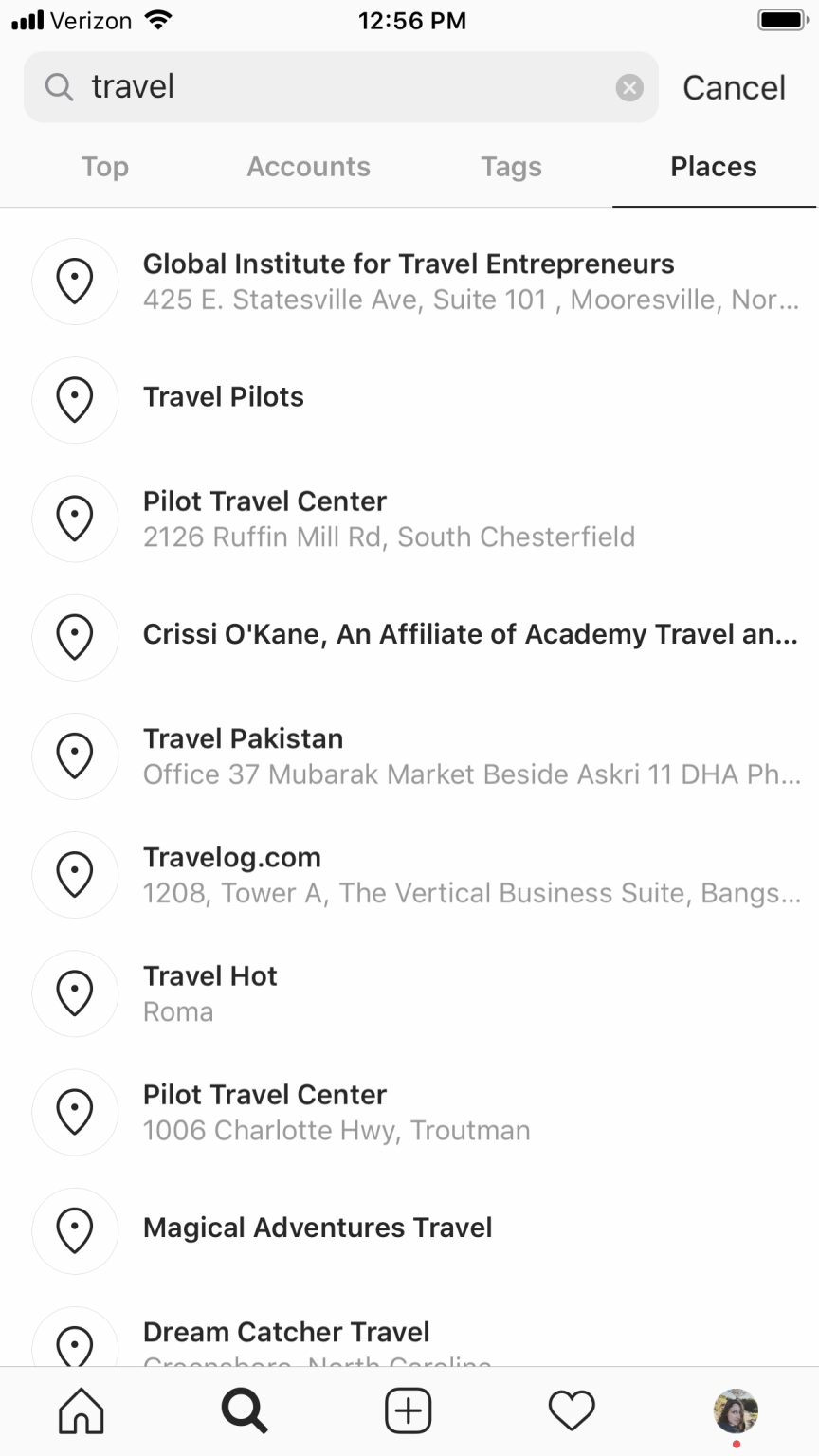The image is a screenshot from a smartphone displaying a search result page. At the top status bar, the carrier is Verizon, it's 12:56 PM, and the battery is fully charged. Just below, there is a search bar with the term "travel" entered. To the right of the search bar is a "Cancel" option. Beneath this are categories labeled "Top," "Accounts," "Tags," and "Places," with the "Places" tab selected.

A list of locations appears under the selected tab, starting with “Global Institute for Travel Entrepreneurs at 425 East Statesville Avenue, Suite 101, Mooresville,” though the address details are cut off. The subsequent locations listed are:
1. Travel Pilots
2. Pilot Travel Center
3. Chrissy O'Kane, an affiliate of Travel Academy
4. Travel Pakistan
5. Travelog.com (spelled T-R-A-V-E-L-O-G.com)
6. Travel Hot
7. Another Pilot Travel Center
8. Magical Adventures Travel
9. Dream Catcher Travel

At the bottom of the screen, navigation icons are visible, including: a home button, a search icon, an "add a location" button, a heart for favorite locations, and the user’s profile picture on the bottom right.